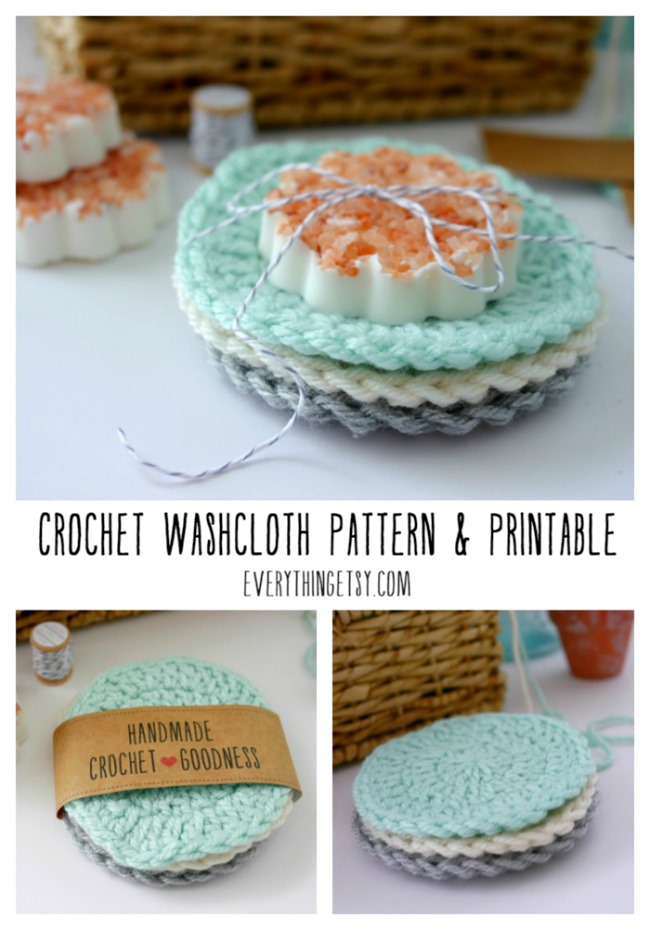This image is a detailed promotional flyer for handmade crochet washcloths, targeted at small business advertising on Etsy. The flyer is divided into three panels with centrally placed text that reads, "Crochet Washcloth Pattern and Printable at EverythingEtsy.com." The top half of the flyer shows a bundle of three crochet washcloths in light blue, white, and dark blue, neatly tied together with a striped blue and white string. Placed on a white surface with a wicker basket visible in the background, this section also features a bar of soap. The bottom half of the flyer contains two smaller images: one on the left displaying the bundled crochet washcloths with packaging labeled "Handmade Crochet Goodness," and one on the right showing another arrangement of the washcloths in a circular pattern, placed next to the same wicker basket. The cohesive color scheme and layout emphasize the product's handcrafted quality and aesthetic presentation.